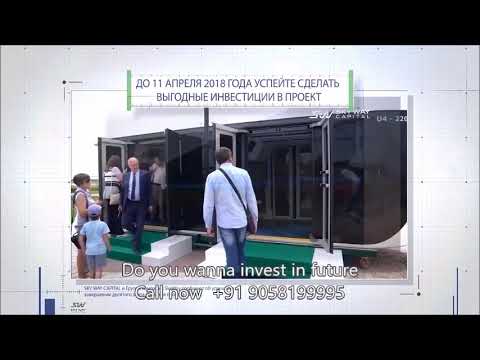The image depicts a still from an international commercial, possibly promoting real estate or modular homes, situated in a foreign country. It features a predominantly white background with a black border at the top and bottom. At the center of the scene, there is a small, shipping-container-like structure with windows and doors, possibly resembling an instant house.

The structure has two doors, each accessible via white steps covered with green carpet. A man dressed in a blue suit with a tie is descending one of the staircases, while another man in blue jeans and a dress shirt, carrying a satchel, is facing away from the camera. Additionally, a woman and a child appear to be looking up at the building.

The top of the image features some text written in a foreign language that might be Russian or Slavic, adding an international context. Below the structure, a prominent English caption reads, "Do you want to invest in the future? Call now." It is followed by an international phone number starting with +91, indicating an Indian dialing code: +91905819995. The sky above is a dull grey, contributing to an overcast ambiance.